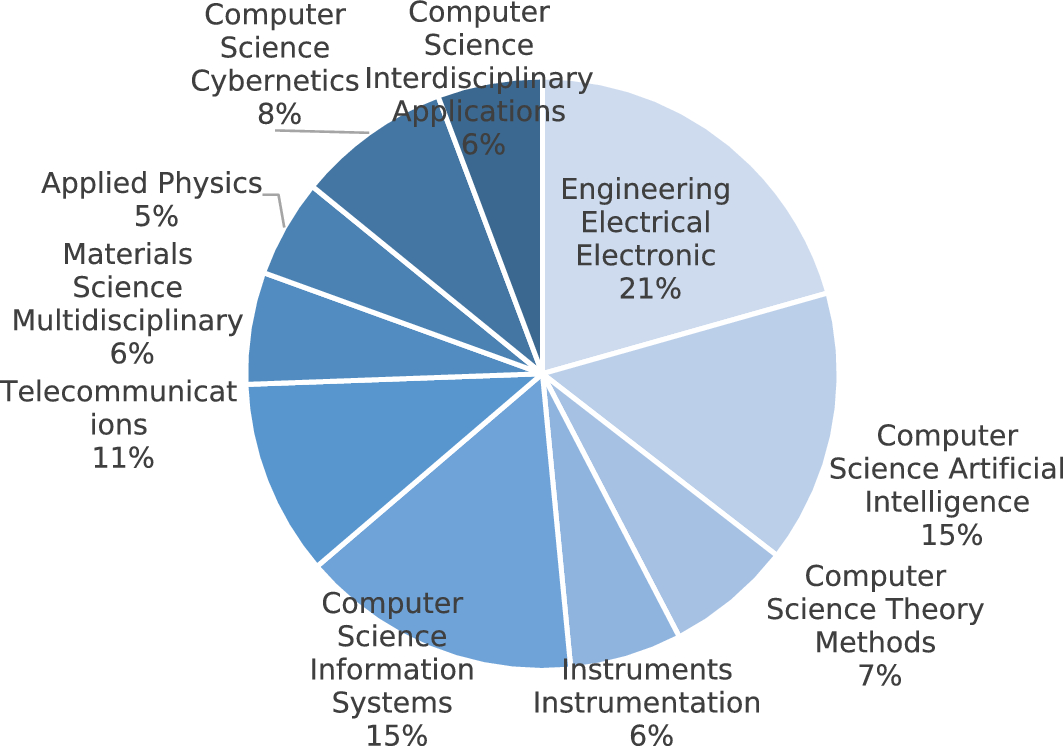The image is a contemporary and eye-catching pie chart that effectively breaks down the percentages of different types of studies or disciplines, likely related to computer science, engineering, and related fields. The chart is divided into 10 sections, each shaded in varying shades of blue from dark to light, starting with the darkest blue at the top left and gradually transitioning to the lightest blue at the top right. 

The sections are labeled clearly with their respective disciplines and percentages. The largest segment, occupying 21% of the chart and shaded in dark blue, represents "Engineering, Electrical, Electronic." The next significant portion, in light blue, depicts "Computer Science, Artificial Intelligence" at 15%. Other notable sections include "Telecommunications" at 11%, "Computer Science, Information Systems" at 15%, and "Computer Science, Cybernetics" at 8%.

Smaller sections include "Computer Science, Theory Methods" at 7%, "Instruments, Instrumentation" at 6%, "Material Science, Multidisciplinary" at 6%, "Applied Physics" at 5%, and "Computer Science, Interdisciplinary Applications" also at 6%.

The pie chart is designed with white dividing lines to distinctly separate each section, making it not only informative but also visually appealing—suitable for display in textbooks, posters, or classroom walls.